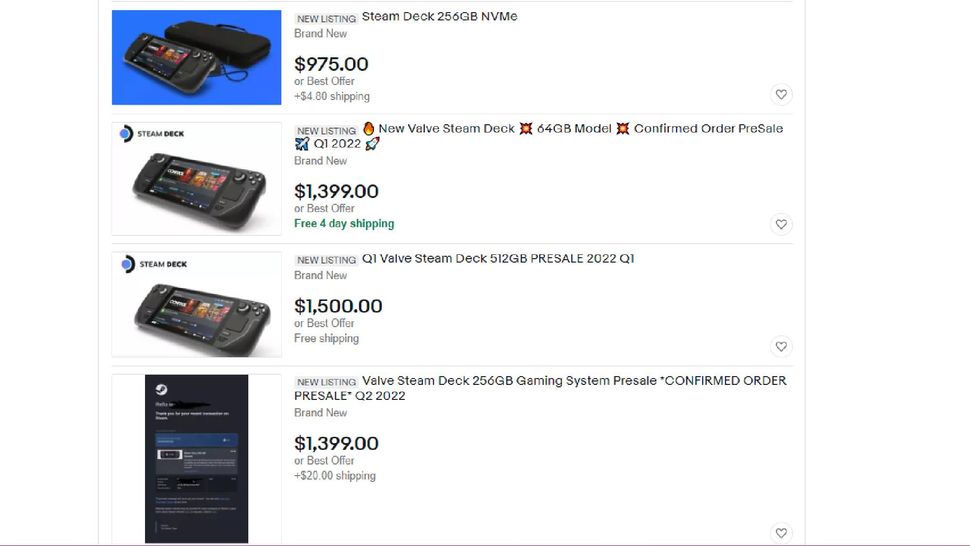This is a screenshot of a shopping webpage featuring four listings for the Steam Deck video game system, each offering different models and prices:

1. At the very top, the first listing showcases a "New Listing: Steam Deck 256GB NVMe," described as brand new and priced at $975 or best offer, with an additional $480 shipping fee. The listing includes an image of the Steam Deck set against a blue background.

2. The second listing below is titled "New Listing: New Valve Steam Deck 64GB Model, Confirmed Order Pre-Sale, Q1 2022." It is brand new, available for $1,399 or best offer, with free $40 shipping. The accompanying image features the Steam Deck with a white background.

3. The third listing, "New Listing: Q1 Valve Steam Deck 512GB Pre-Sale, 2022," offers a brand new unit for $1,500 or best offer, with free shipping. This listing also includes an image of the Steam Deck against a white backdrop.

4. The fourth and final listing is presented as "New Listing: Valve Steam Deck 256GB Gaming System Pre-Sale, Confirmed Order Pre-Sale, Q2 2022." Priced at $1,399 or best offer, it includes a $20 shipping fee. The image provided appears to be a screenshot from the official Steam webpage, presumably displaying the Steam Deck.

Each listing highlights a different configuration and shipping detail, offering potential buyers various options to choose from.